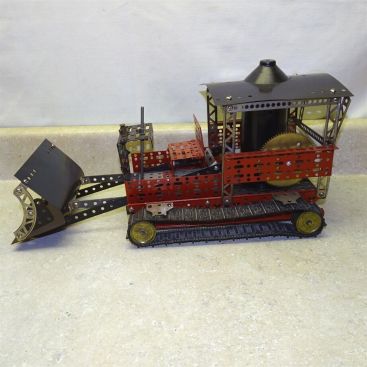In the image, there is a detailed and intricately handmade model of an old-timey bulldozer, reminiscent of 1920s machinery. The bulldozer, prominently positioned at the center of the image, is placed on a white surface against a light bluish-gray background that suggests the setting is within a room in a house. The bulldozer's cab is distinctive with an open design, lacking windows, and surrounded by red railings. The overall construction features a mixture of colors: black tracks, reddish-brown railings, copper-colored wheels and gears, and a black bucket adorned with copper-colored embellishments. It evokes the appearance of aged construction equipment, possibly used for picking up materials like sand. The model is detailed with materials including metal, and the wheels within the tracks are highlighted in yellow. There is no text in the image, which showcases this singular, nostalgic item against a minimalist backdrop.